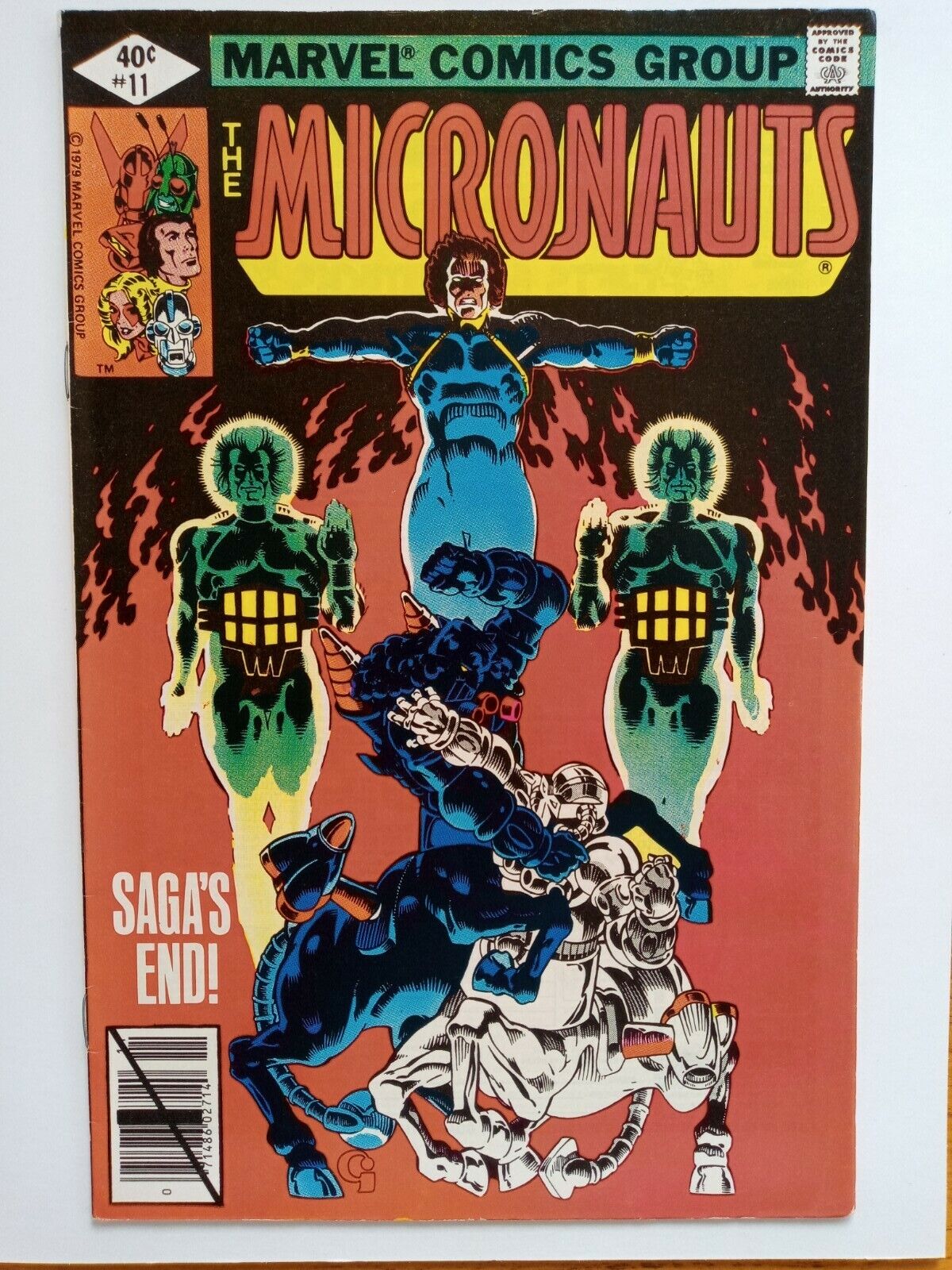This is a cover photo of a vintage Marvel Comics issue from 1979, featuring The Micronauts. At the very top, it reads "Marvel Comics Group," accompanied by the "Approved by Comics Code Authority" seal. This is edition number 11, priced at 40 cents. The prominent main heading says "The Micronauts" with the subtitle "Saga's End" depicted. Dominating the center is a fierce-looking blue character with muscle tone, staring directly out from the image. Flanking this figure are two green, human-like twins with radiated appearances, showcasing green skin and yellow legs. Below, a dramatic battle scene unfolds with two demon-like horses: one white and one black, set against a striking red background.